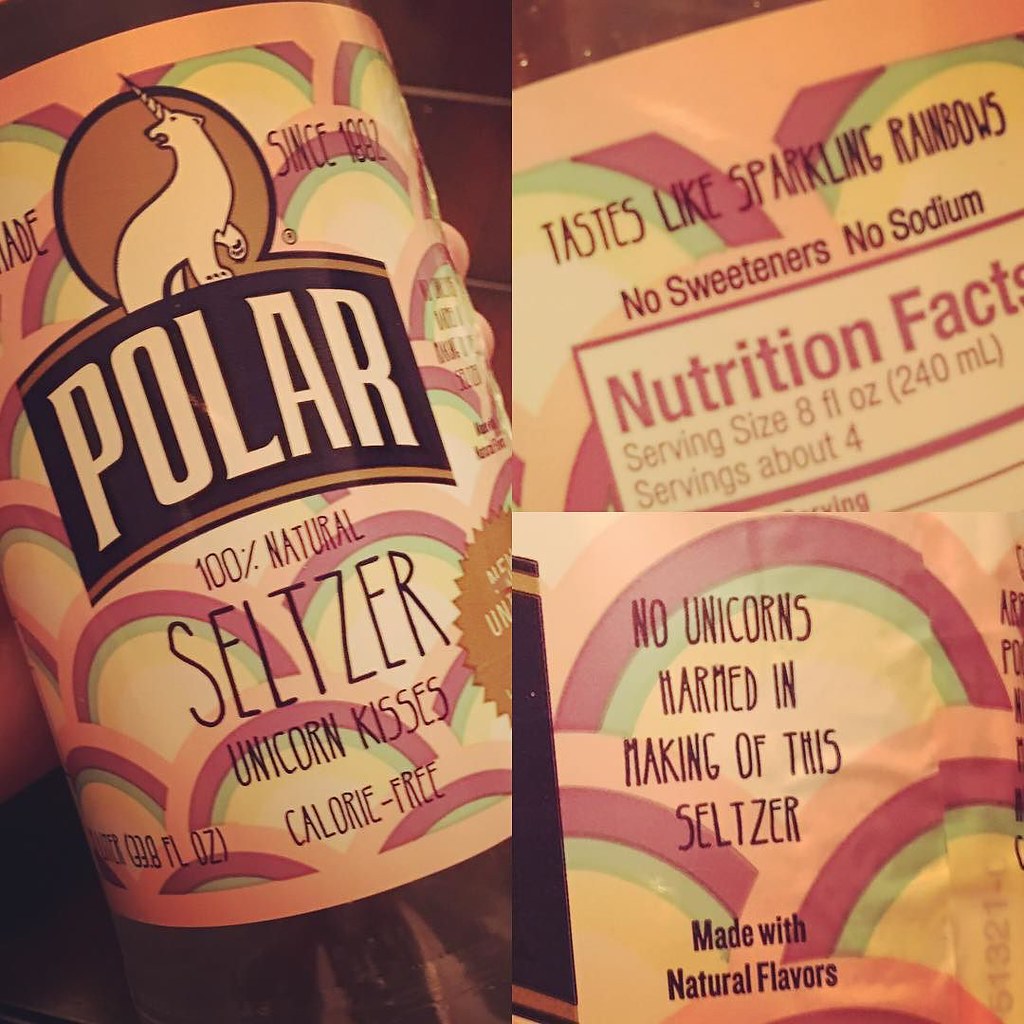The image is a composite photograph consisting of three framed sections depicting a colorful seltzer or ice cream container. On the left-hand side, there is a large main image taking up the entire section, showing someone holding a vividly decorated container with light pink, purple, and green fish scale-like patterns. Prominently displayed on the container is a circular emblem featuring a polar bear with a unicorn horn, set against a brown circle with a black outline. Below the emblem, the word "POLAR" is written in bold white capital letters on a black background with brown borders. The container also includes phrases such as "100% Natural Seltzer," "Unicorn Kiss," and "Calorie Free."

The right-hand side is divided into two smaller images stacked vertically. The top image contains text advertising the product: "Tastes Like Sparkling Rainbows," "No Sweeteners," and "No Sodium," alongside the nutritional facts which state a serving size of 8 fl oz (240 ml). The bottom image provides a playful disclaimer: "No Unicorns Harmed in the Making of this Seltzer," with a note that it is made with natural flavors. The overall lighting suggests the photographs were taken indoors, as the images appear somewhat washed out.